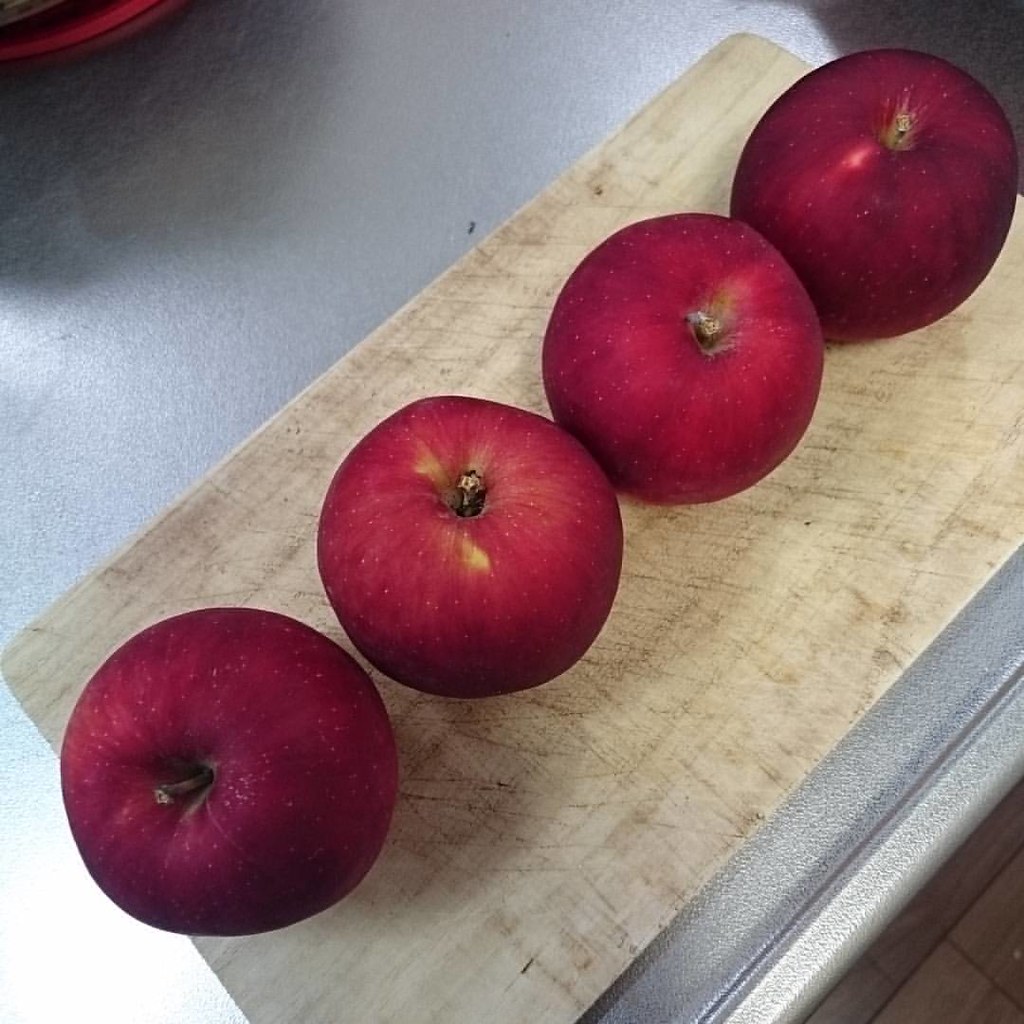The image depicts four dark red apples, each resembling a rich burgundy hue with occasional plum and purple tints, lined up in a neat row. They rest on a well-worn, light-colored wooden cutting board bearing visible cut marks, signifying extensive use. The cutting board is set upon a metallic steel tabletop that adds a modern contrast to the rustic board. The apples, uniform in size, are nearly touching and glisten subtly, with brown stems pointing upwards. Flecks of yellow and green can be seen near the stem area, and some white specks dot their otherwise richly colored skins. The perspective of the photo offers a top-down view that captures these details meticulously.